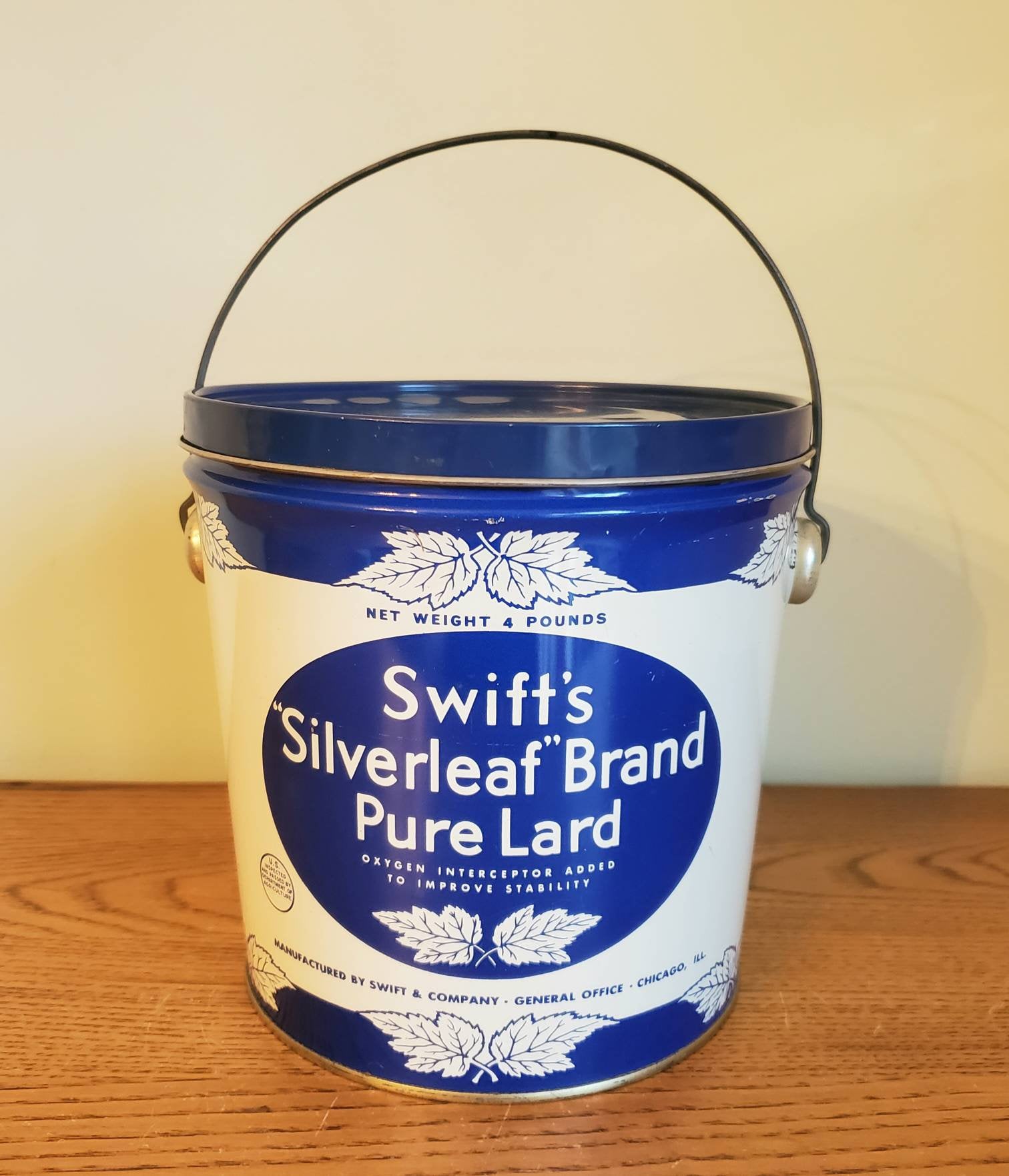This detailed photograph showcases a vintage Swift's Silverleaf brand pure lard tin bucket, prominently displayed against a white wall with a subtle yellow hue. The bucket is metallic, predominantly white with blue accents including the lid, base, and various decorative elements. Centered on the tin is a distinctive blue circle adorned with white lettering and leaf outlines, reading "SWIFT Silverleaf brand pure lard" with the added note "oxygen interpreter added to improve stability." Additional details on the tin include "Manufactured by Swift and Company, General Office, Chicago, Illinois" and "net weight 4 pounds" prominently displayed at the top. The bucket’s handle is upright, contributing to its classic look. It is positioned on a basic credenza or table, providing a neutral backdrop that emphasizes the bucket's design and nostalgic appeal.